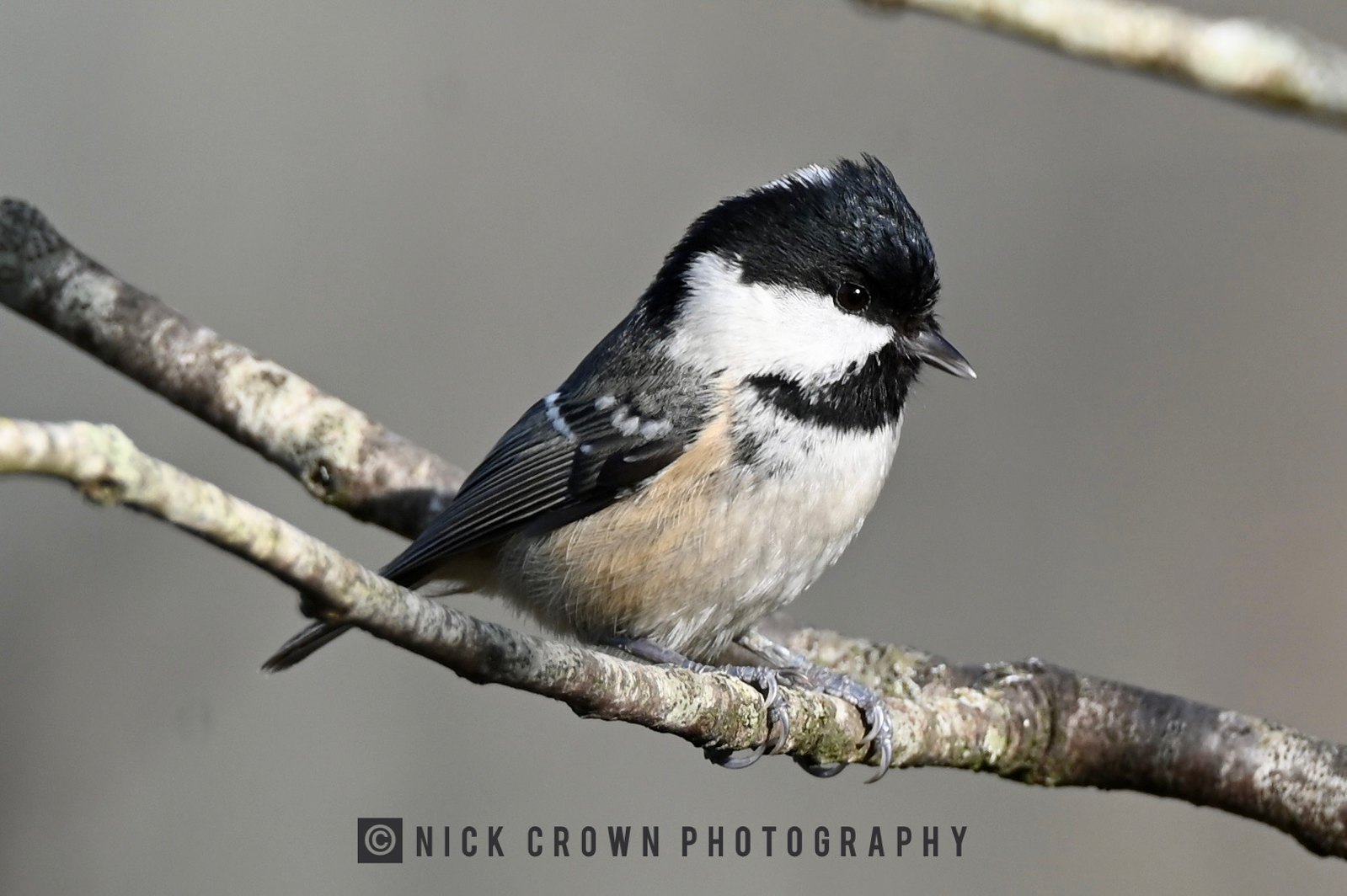In this extreme close-up, professional photograph by Nick Crown Photography, a small bird, likely a chickadee, is perched on a forked tree branch that spans the entire width of the image. The bird's feet are tightly clasping the branch, with another blurred branch visible in the upper right corner. The background is artistically blurred, highlighting the bird's intricate details. It has a short, dark gray beak, black feathers on top of its head forming a crest, and similarly black feathers on its throat and wings. The bird’s eyes blend into the black crest, making them almost indiscernible. Stark white feathers adorn its face, wrapping around from beneath its eye to its cheek. Its belly showcases a mix of white, tan, and occasional black feathers. The bird appears calm, showing no intention of flight, allowing for a detailed capture of its delicate features and the texture of the branch below it. At the bottom of the image, the text "Nick Crown Photography" marks the photo with a copyright symbol.